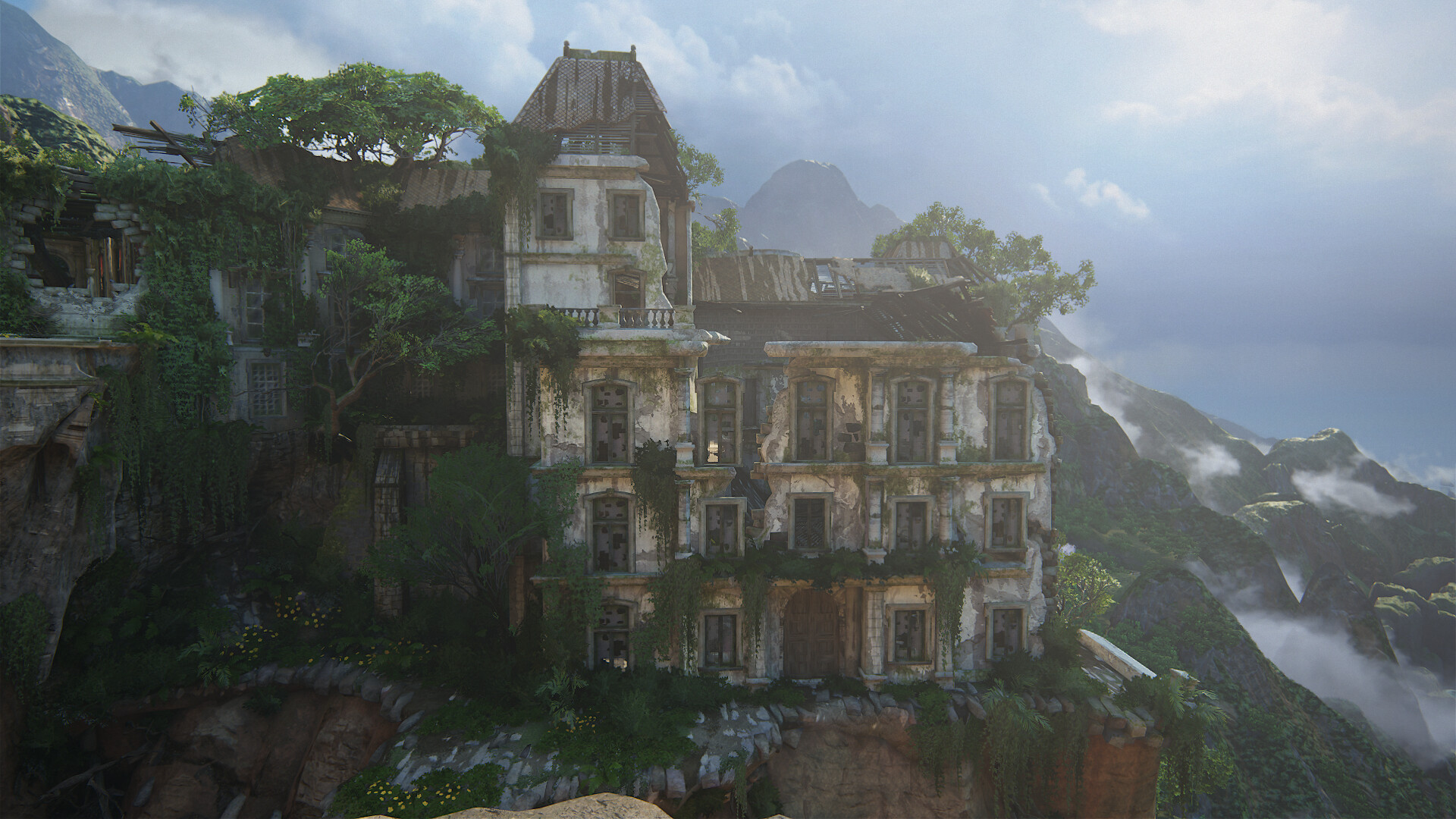This stunning landscape photograph captures a grand, off-white castle seamlessly built into the rugged mountainside. The castle appears weathered and slightly dirty, adding to its ancient, storied charm. Vibrant greenery grows abundantly around the structure and even decorates the windowsills, enhancing its fairy-tale appearance. In the backdrop, the imposing mountains, with a grayish-blue hue, stand majestically, while a light blue sky adorned with scattered white clouds completes this picturesque scene.